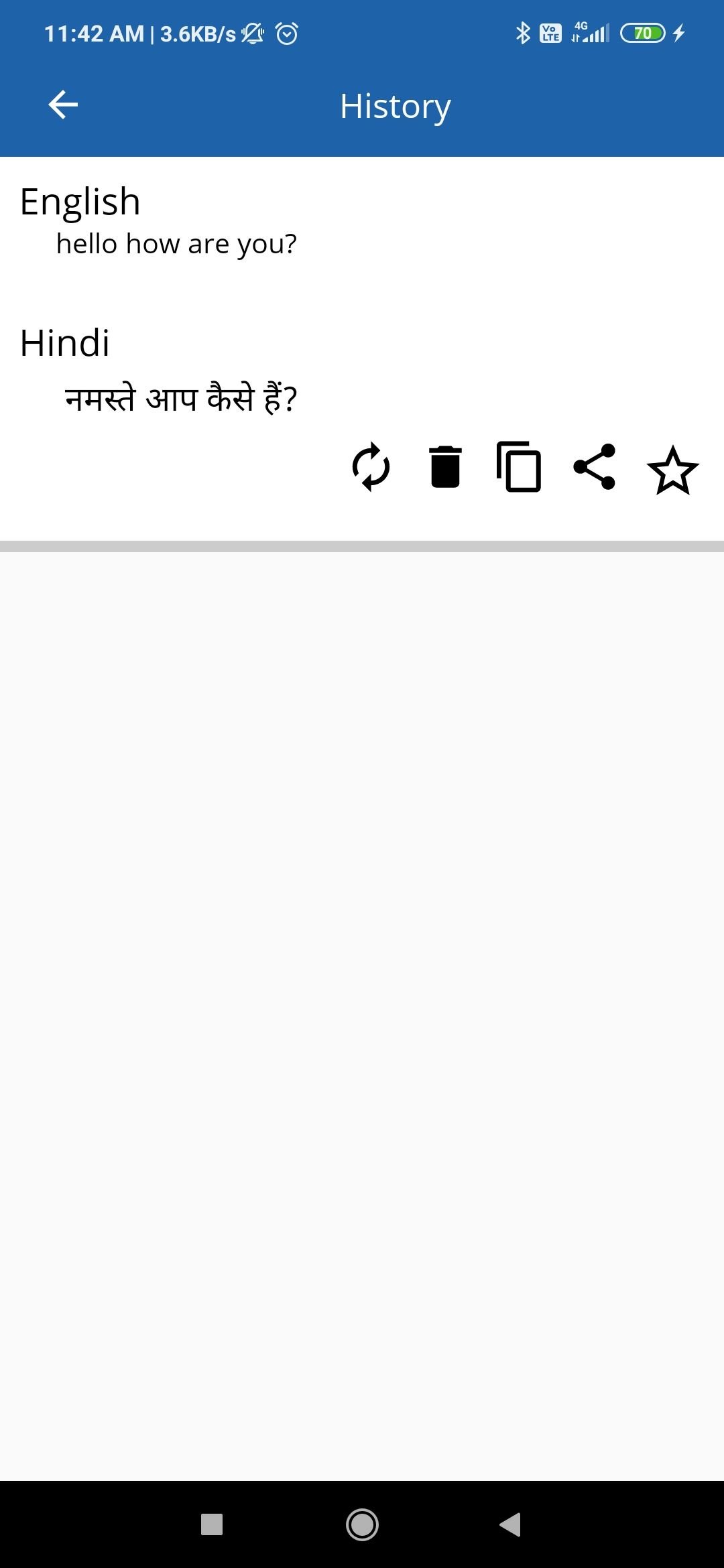The image appears to be a screenshot taken from a smartphone displaying a translation app interface. 

At the top of the image, there is a dark blue status bar. On the left side of this bar, the time reads 11:42 AM. Next to the time, it indicates data usage of 3.6 KB, followed by a "Do Not Disturb" icon and a clock icon. On the right side of the status bar, there is a Wi-Fi icon showing four bars with three filled in, signifying a strong connection. Adjacent to this, a battery icon displays a charge level of 20%.

Below the status bar, a navigation arrow pointing to the left and the word "History" are centrally positioned. The main interface is displayed against a white rectangular background. In the top left corner of this section, the word "English" is shown, indicating the input language. Beneath this, the text "Hello, how are you?" has been typed. Directly below, labeled "Hindi," is the corresponding translated text in Hindi script, presumably also translating to "Hello, how are you?"

To the right of the translated text, there are several icons: a refresh icon, a trash can icon, two overlapping squares symbolizing copy functionality, a share icon depicted as a triangle with three dots, and a star icon for favoriting. A gray horizontal line separates this section from the rest of the screen.

The lower part of the screen consists of an empty gray space extending to the bottom, where a black navigation bar is present. This bar includes three icons: a square symbolizing recent apps, a circle for the home screen, and a left-facing triangle for the back function.